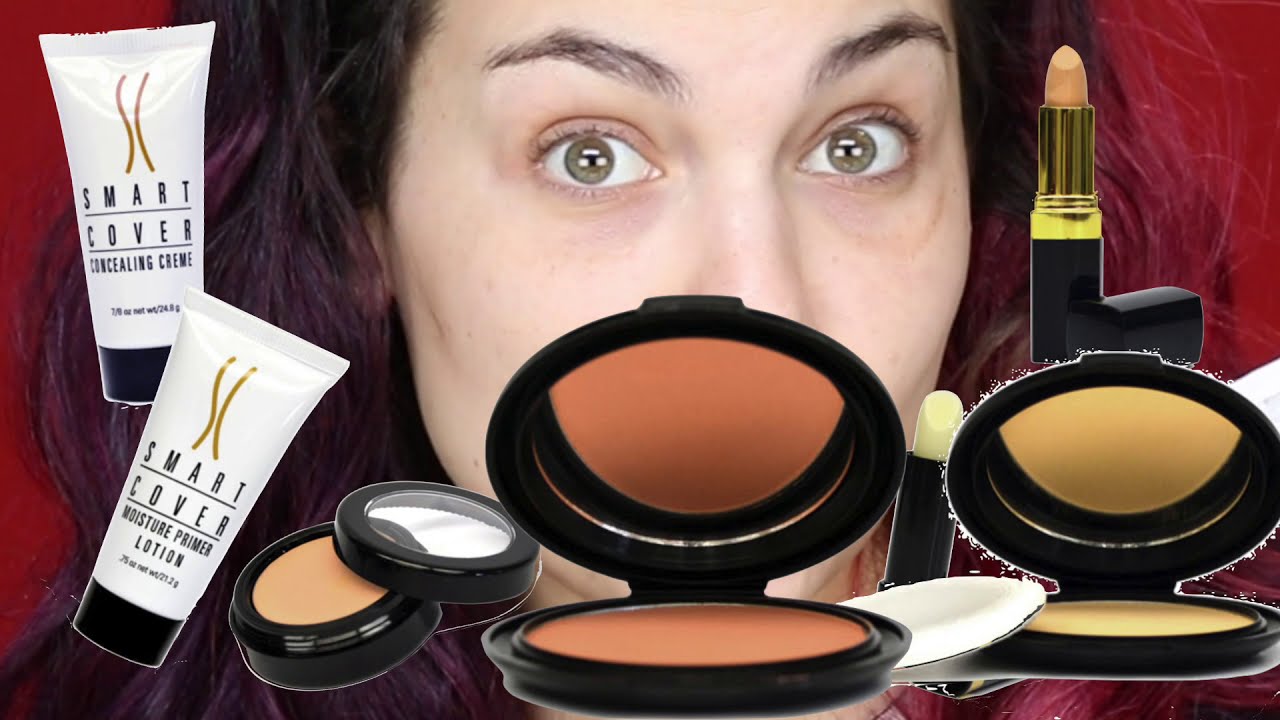In the image, a woman's face takes center stage against a red background, with reddish-brown hair framing her face and extending to shoulder length. She has striking green eyes and a surprised expression, with her eyebrows raised high. The shot is close-up, offering a detailed view of the makeup items spread out in front of her.

In the lower right corner of the image, two compact mirrors reveal peach and yellow blushes. Directly in front of her face sits a black makeup case with brown makeup inside, reflecting its contents in a mirror flipped open above it. To the left, two bottles of lotion labeled 'Smart Cover Concealing Cream' and 'Smart Cover Moisture Primer Lotion,' both in white with black lids, rest side by side.

Propped slightly to the right is another makeup case containing yellow makeup, which reflects prominently in its accompanying mirror. A peach lipstick tube and a black tube with white lipstick are visible on the right-hand side, with the peach lipstick positioned behind her cheek. The red background subtly peeks through on either side of her head, completing the setting focused on this array of beauty products.